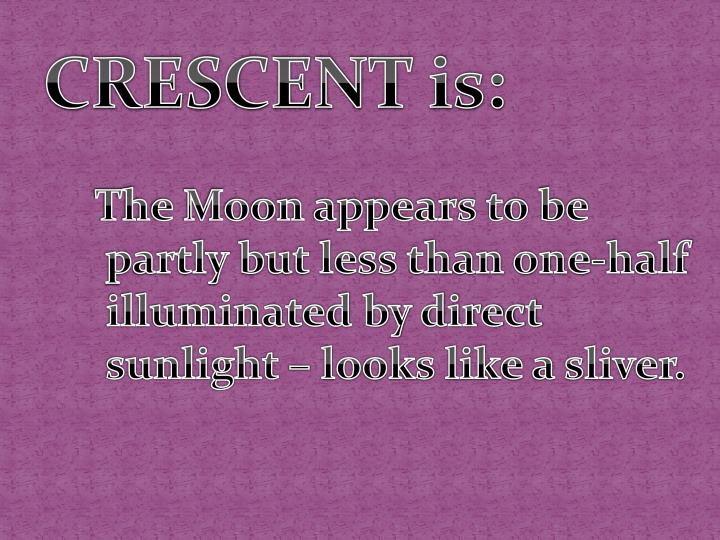The image resembles a PowerPoint slide with a speckled, patterned purple background. Across the top in a bold, black serif font with a white outline reads "CRESCENT IS:". This header is distinctive as each letter is bifurcated with the top half in a lighter gray and the bottom in a darker black color. Below this header, in slightly smaller text positioned centrally, the definition reads: "The moon appears to be partly but less than one half illuminated by direct sunlight—looks like a sliver." Notably, the word "Moon" is capitalized. The overall style and presentation suggest it is meant to be an informative visual slide.